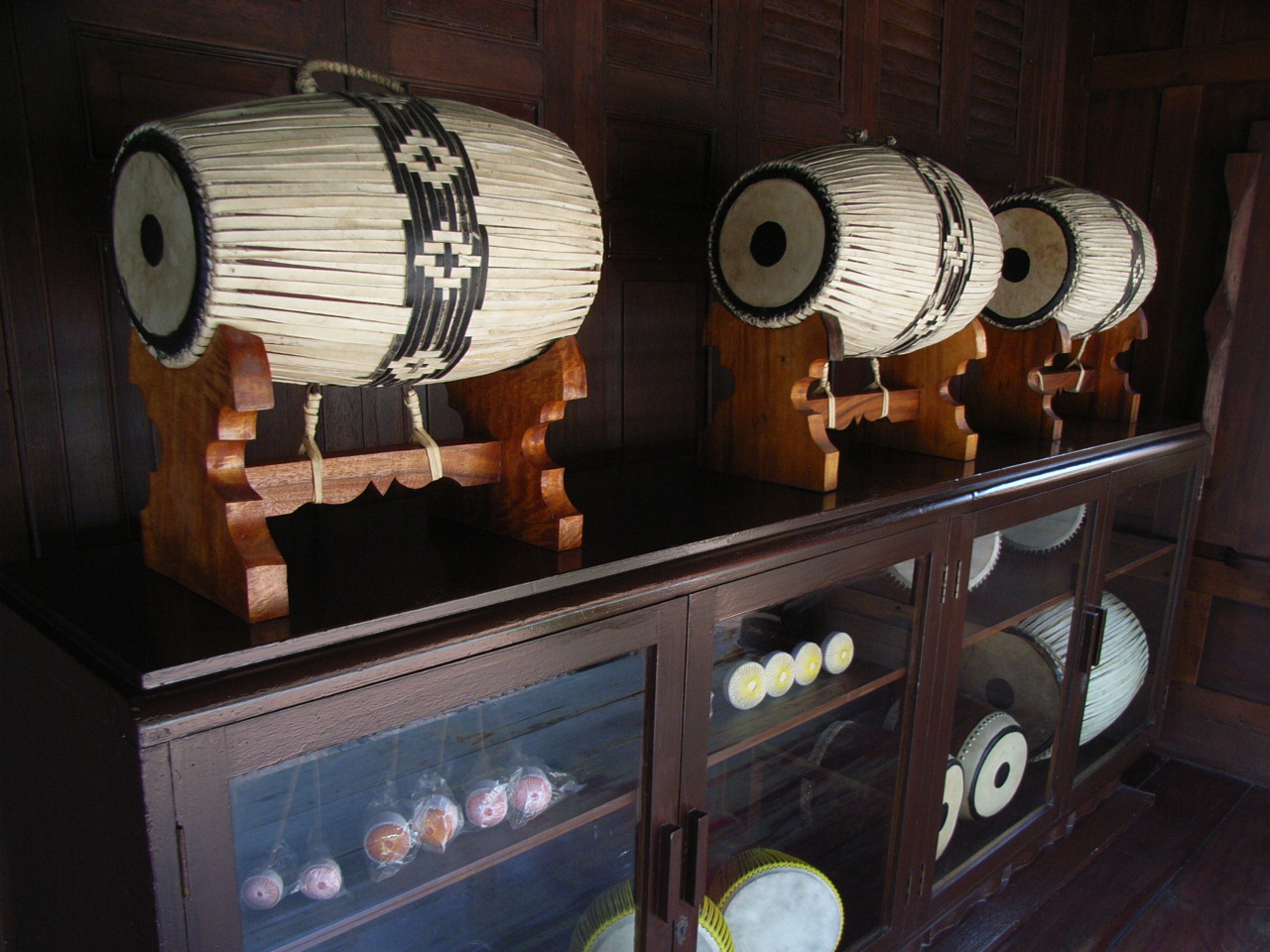The indoor color photograph features a wooden display cabinet, situated at an angle along the bottom left corner, extending towards the middle right side of the image. The case is constructed from dark brown wood with glass-fronted doors, revealing a set of displayed items inside. Although partially cut off, the cabinet consists of four glass-fronted doors, which allow a view of the contents within.

Perched atop the cabinet, resting on wooden stands, are three identical bongo-type drums, laying on their sides. These drums are crafted with a rough, white material resembling packaging strips, oriented vertically from top to bottom when upright. Encircling their middle is a black strip adorned with geometric patterns of white diamond cutouts and a central black plus icon. The drum heads feature a black line around their circumference and a central black dot.

Inside the cabinet, a shelf runs along the top third, though it is unclear if it spans the entire width or is divided into sections. On the bottom shelf of the case, there are several larger bongo-type drums. Additionally, in the top-left section of the leftmost compartment, a pair of drumsticks is visible through the glass, positioned with the striking ends facing outward and the handles angled back. The display case serves as an elegant showcase for these intricately designed musical instruments.